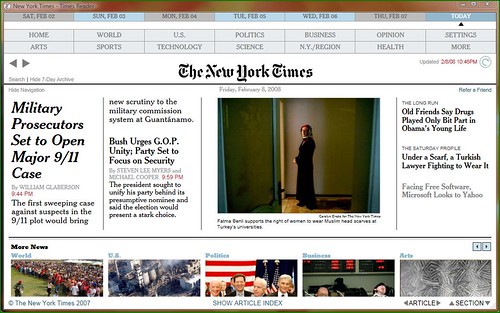The webpage is from the New York Times, featuring an array of articles and images. The top of the page displays the New York Times logo prominently in the center, set against a black background. Above the logo, there are navigation categories in gray, which include U.S., Politics, Science, Business, World, Sports, Home, Arts, Settings, More, Health, and Opinion.

Beneath the navigation bar, the headline "Military Prosecution Set to Open Major 9/11 Case" is prominently featured, signaling a significant article. Another bold headline reads, "Bush Urges GOP Unity Party Set to Focus on Security."

An image is displayed on the page showing a person clad in a black robe with red hair, seemingly looking out of a window. Below this image, the text reads: "Old friends say drugs played only a bit part in Obama's young life."

The lower section of the webpage features a series of cropped images from around the world. One image shows a large crowd, possibly viewing a professional golf game. Another image, characterized by blue and gray tones, is difficult to discern. A third image shows world leaders standing in front of an American flag. The next image depicts two individuals, and the final image in the series is composed of gray and white hues.

Overall, the webpage is a typical layout for the New York Times, combining significant news headlines with visual elements to captivate readers.